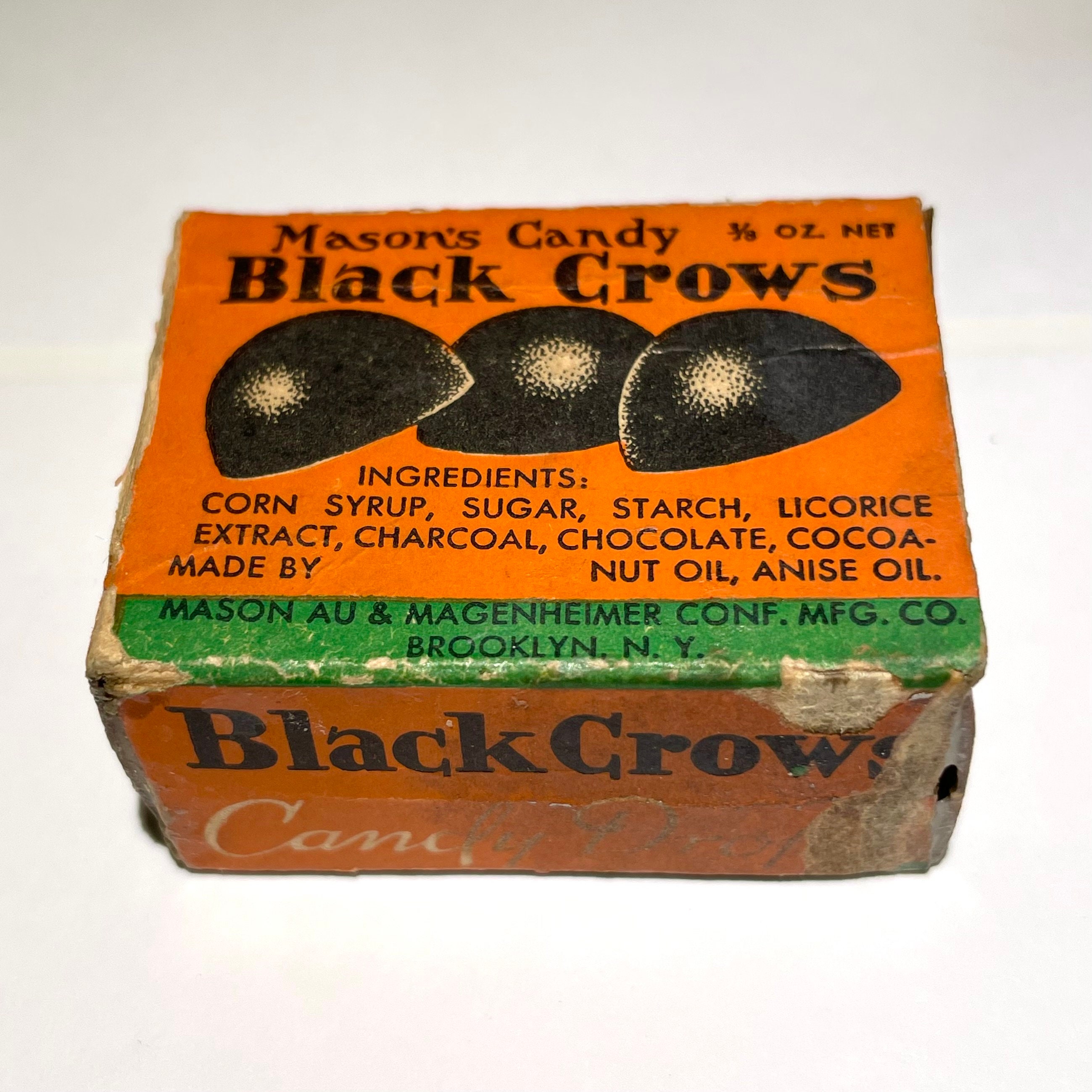This image displays a close-up of a tattered vintage box of Mason's Candy Black Crows. The box, featuring an orange and green border with black lettering, appears square and visibly worn, with its corners showing signs of wear and some parts partially caved in. The front of the box prominently shows little pictures of what seem to be gummy candy shaped like black crows. The text on the orange box reads "Mason's Candy" at the top and specifies "Three-eighths ounce net." It also reads "Black Rose" and lists the ingredients: corn syrup, sugar, starch, licorice extract, charcoal, chocolate, cocoa, nut oil, and anise oil. Additionally, the manufacturer's details are provided on a small green label, indicating "Mason AU and Magenheimer Conf MFG Co., Brooklyn, New York." Despite its aged and fragile appearance, the box carries a nostalgic charm, emphasizing its vintage nature.